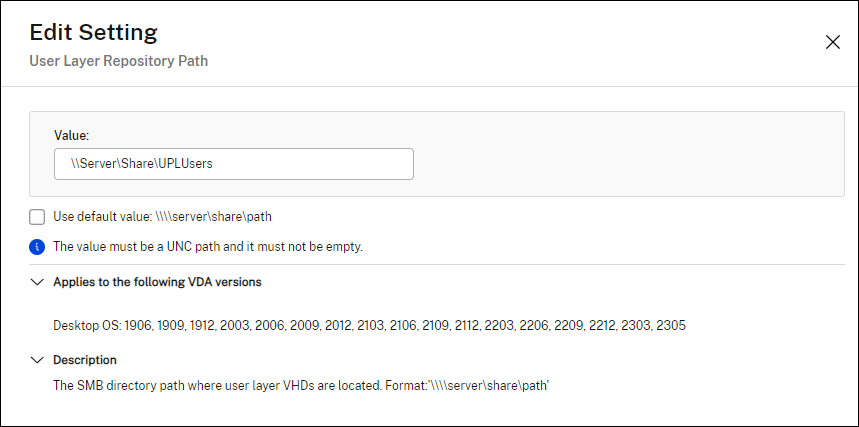"Detailed screenshot displaying server configuration settings. The screen shows a section titled 'Edit Setting: User Layer Repository Path.' On the right-hand side, there is an 'X' icon. Below this icon, the label reads, 'Value: \\Server\share\upl\users\user (User Default).' The notice indicates that the value must be a UNC path and cannot be empty. This setting applies to specific VDA versions and involves defining the SMB directory path where user layer VHDs are located. The entire interface is presented on a white background with black text."